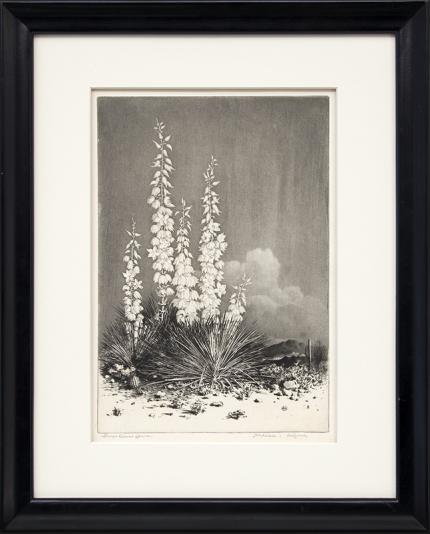This is a photograph of a black-framed, meticulously matted black and white illustration or photograph from an old book of plant life, prominently featuring a magnificent yucca cactus in bloom. The frame has a double matting, with a larger white mat nestled inside the black outer frame, giving the artwork an enhanced depth and a striking contrast. The yucca cactus, situated amidst a barren landscape of sand and rocks, stands tall with its flowering stalks reaching up to three or four feet. The blooms are depicted with white flowers or seed sacks, radiating a crisp brightness that starkly contrasts the grayscale background. The scene captures a desolate desert landscape, with a few scattered pebbles at the base of the cactus and an expansive, grayed-out sky. In the distance, there is a hint of low mountains and ethereal clouds, providing a sense of vastness and isolation to the composition. The careful framing and detailed depiction capture the raw, natural beauty of the yucca in its arid habitat.